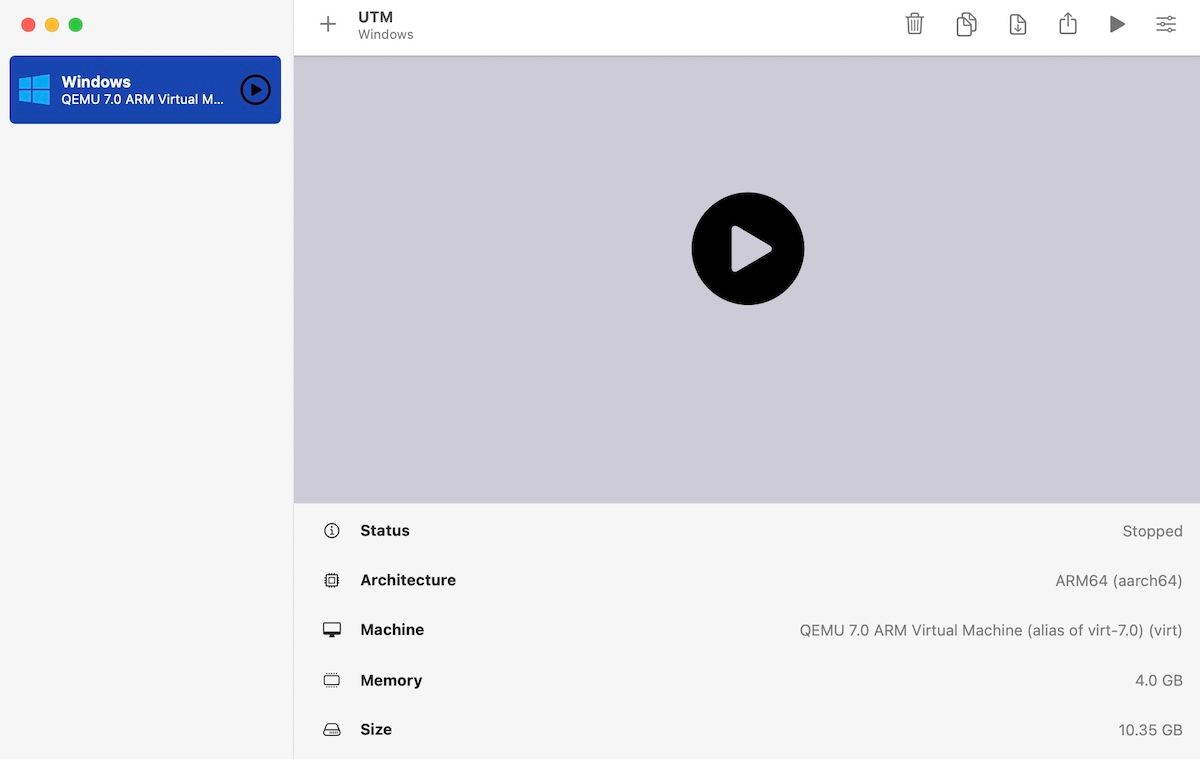The image showcases a Windows program interface with detailed elements. On the left side of the display, there's a partial view of the blue Windows emblem adjacent to the text "Windows QEMU 7.0 ARM Virtual," which is partially cut off. The text appears to be clickable and has been selected, as indicated by its blue highlight. 

To the right, a section labeled "UTM" features a lilac screen with a central black button prompting the user to "click to start the video." 

Below this display, there is a vertical list that includes status, architecture, machine, memory, and size, each accompanied by corresponding icons on the left. The status is marked as "stopped," the architecture is specified as "ARM64" (AARCH64), and details about the machine number, memory, and size follow in respective order.